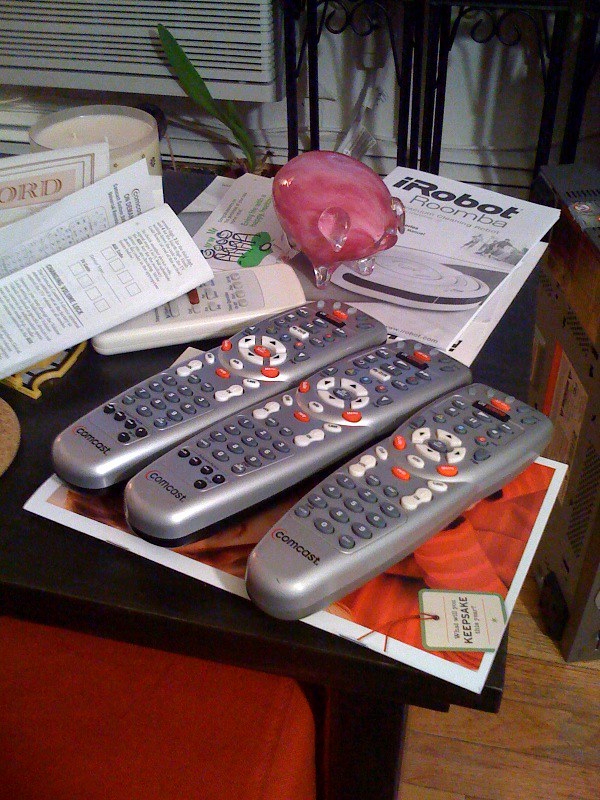This color photograph captures a cluttered corner of a living space dominated by a dark wooden coffee table. Centrally positioned on the table are three gray Comcast cable remote controllers, distinguished by their orange, white, and black buttons. These remotes are arranged neatly on top of an orange and white placemat. Surrounding these remotes are various items, contributing to the disarray. Towards the upper part of the table, there's a manual for an iRobot Roomba, partially covered by a small, ornate pink glass figurine resembling a pig. Flanking the remotes on the left is a smaller, white remote, presumably for an air conditioner, situated near a white candle. Scattered around are other leaflets and pamphlets, adding to the sense of clutter. The backdrop of the scene includes a chair, an air conditioning unit visible in the upper left corner, and a gray wall, blending into the overall composition. The floor beneath the table transitions from a red carpet on the left to a brown wooden floor on the right, framing the coffee table's chaotic surface.